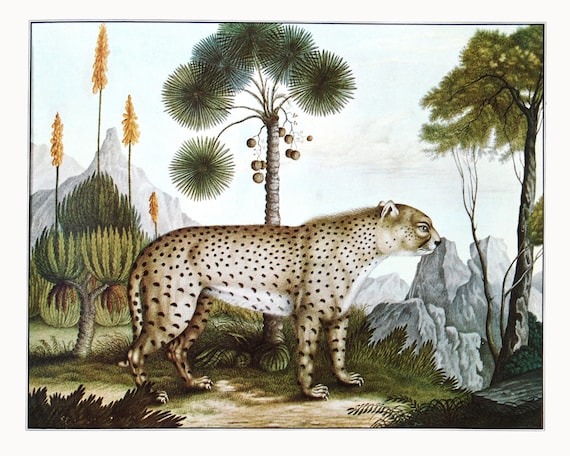This intricate, flat painting, reminiscent of an Indian or Asian style, vividly depicts a heavily stylized big cat, possibly a leopard, cheetah, or jaguar, in a lush, fantastical jungle setting. The cat, viewed from the side, has a stocky, muscular build and a coat of pale beige with distinctive black spots. Its tail hangs down as it stands watchfully on a rugged, rocky landscape. Surrounding the feline is a diverse array of exotic and spiky vegetation, including a striking palm tree with spherical palmate leaves and large coconuts, alongside a peculiar fern-like plant with golden banana-like growths. In the backdrop, muted, grayish mountains loom under a craggily cliff edge, creating a subdued, almost monochromatic contrast to the slightly yellowish and olive-green tones of the greenery. The painting features no text or artist's signature, adding to its enigmatic, old-world charm, evocative of scientific illustrations from the 1700s or 1800s.